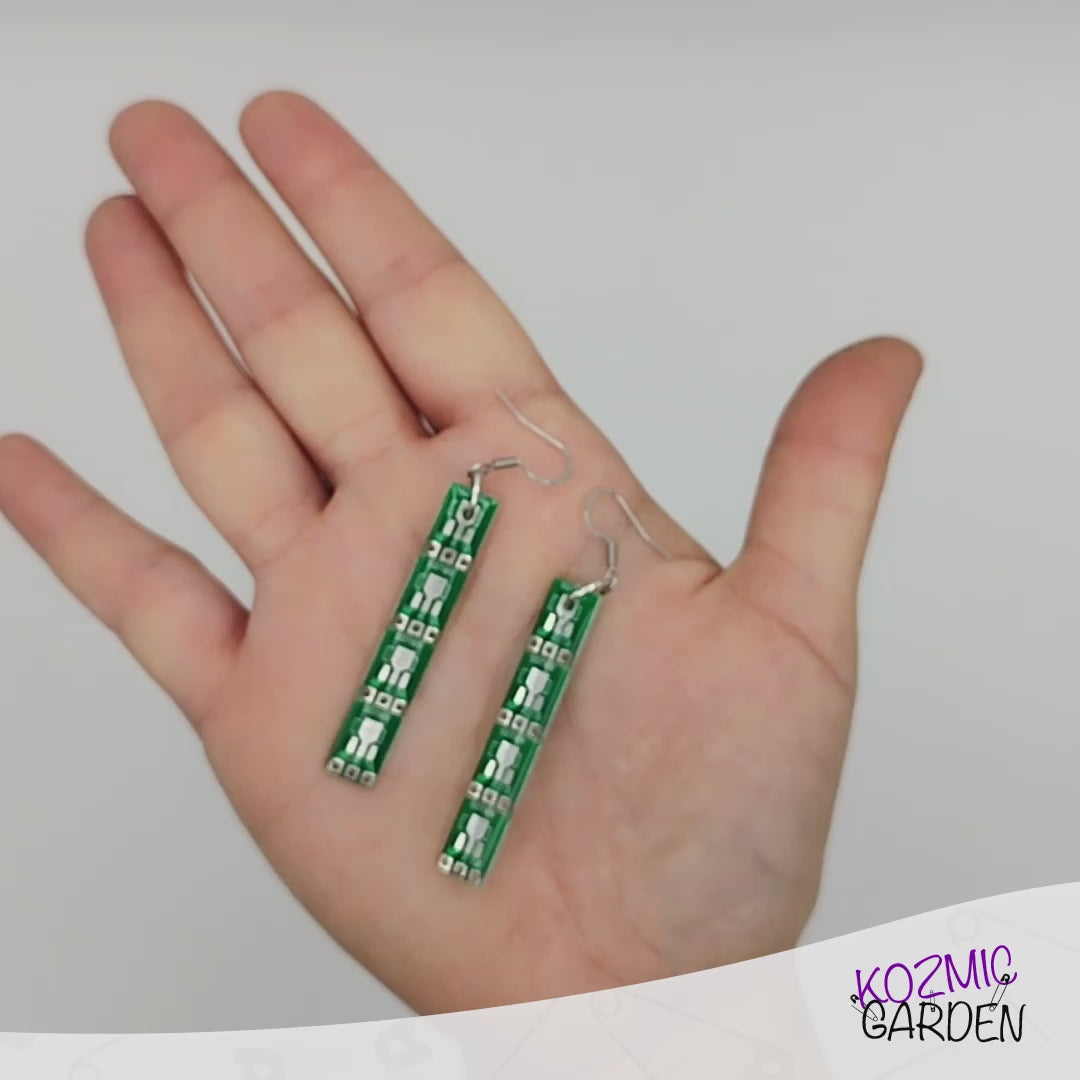In the image, there's a close-up, slightly low-quality photograph of a small white child's left hand, held with the palm facing leftward and the thumb pointing upward. The hand is gently cupping a pair of green drop earrings, which resemble circuit boards encased in resin with silver hooks and intricate designs that could be patterns or letters such as "AOC" or "00C". A light-to-medium gray background fills most of the photo, transitioning to a lighter gray or almost white area at the bottom. In the lower right corner, the unique logo of Cosmic Garden—spelled "K-O-Z-M-I-C" in purple, with "Garden" in black—appears, with safety pins cleverly connecting the two words.